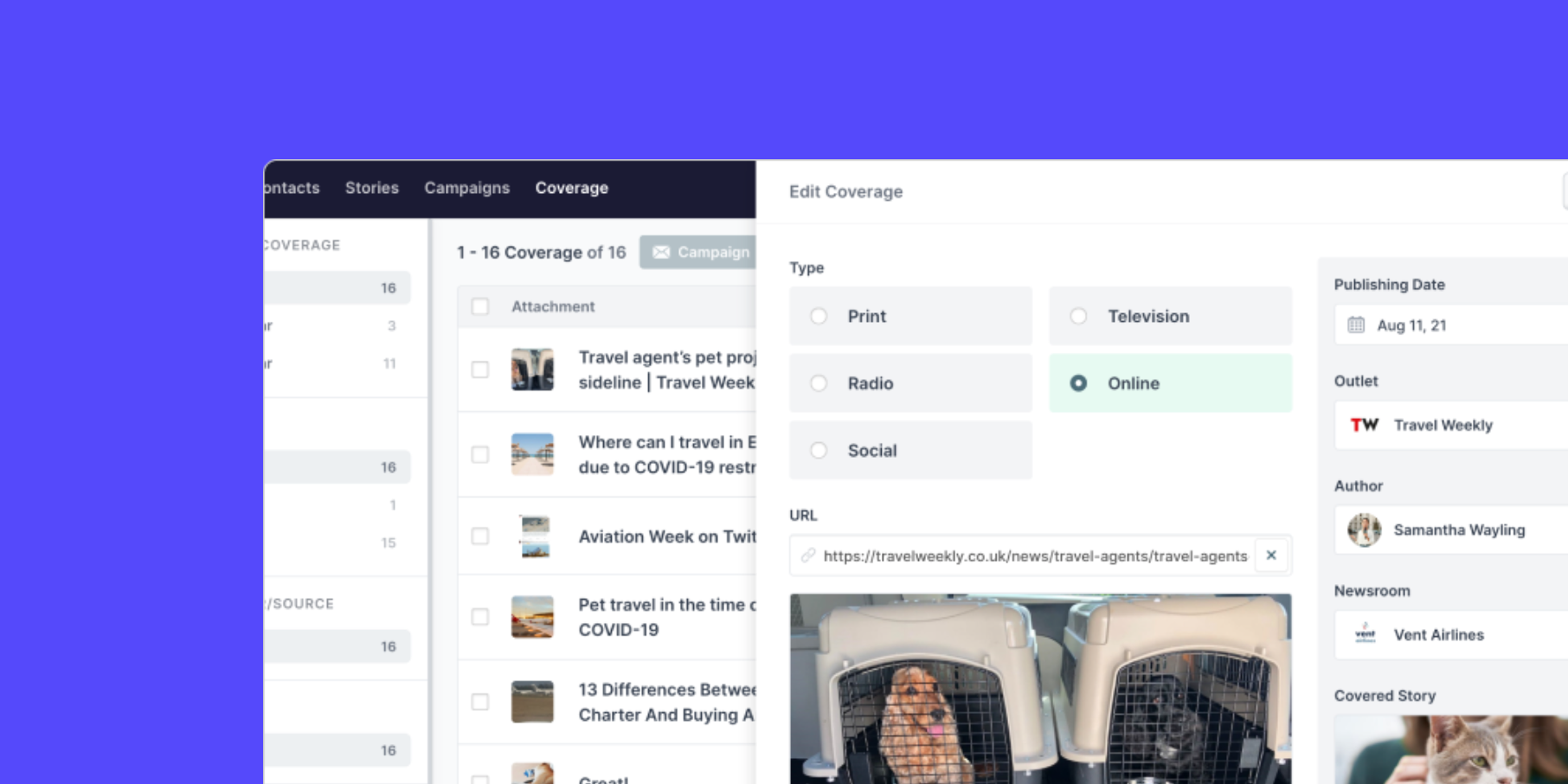Here is a cleaned-up and detailed caption for the described image:

---

**Caption:**
A cropped screenshot depicts a user’s computer screen featuring two windows open against a blue wallpaper background. The wallpaper forms an "L" shape, with the main portion occupying the top of the screen and a smaller section extending down the left-hand side.

The background window appears to be a webpage from a travel site, possibly designed to help users find pet-friendly travel options during COVID-19. The site features a navigation bar at the top left, with menu items labeled "Contacts," "Stories," "Campaigns," and "Coverage." The "Coverage" tab is highlighted, indicating this section is currently selected.

On the left-hand side of the travel webpage, although the specific text is unclear, there are likely filters or search criteria related to coverage options. On the right-hand side, there's a note indicating "1 out of 16," suggesting there are multiple search results or coverage options available for the criteria entered.

Hovering in front of this window is another webpage providing various options related to the search results from the initial site, including URLs for online resources. The juxtaposition of these windows emphasizes the user's effort to explore travel possibilities that accommodate pets amid pandemic restrictions.

---